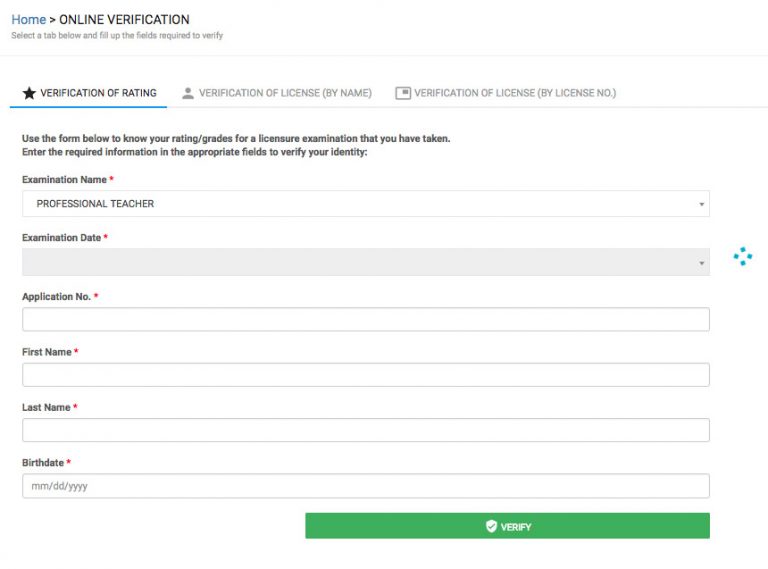In the upper left-hand corner of the image, there is the word "HOME" displayed in blue-dot lettering, followed by the greater-than symbol and then the capitalized words "ONLINE VERIFICATION." Below this, it instructs, "Select the tab below and fill in the required fields to verify," separated by a horizontal gray line.

There are three categories displayed from left to right as follows:
1. A star emoji next to the text "Verification of Rating."
2. A person emoji next to the text "Verification of License (by Name)."
3. An ID card emoji next to the text "Verification of License (by License Number)."

The selected tab is "Verification of Rating," and it states the following: "Use the form below to know your rating/grades for a licensure examination that you have taken. Enter the required information in the appropriate fields to verify your identity."

The form contains several fields:
- "Examination Name" (required) where the user has filled in "Professional Teacher."
- "Examination Date" (required) which is currently grayed out.
- "Application Number" followed by a red mandatory star emoji.
- "First Name" followed by a red star.
- "Last Name" followed by a red star.
- "Birth Date" followed by a red star with the format indicated as MM/DD/YYYY.